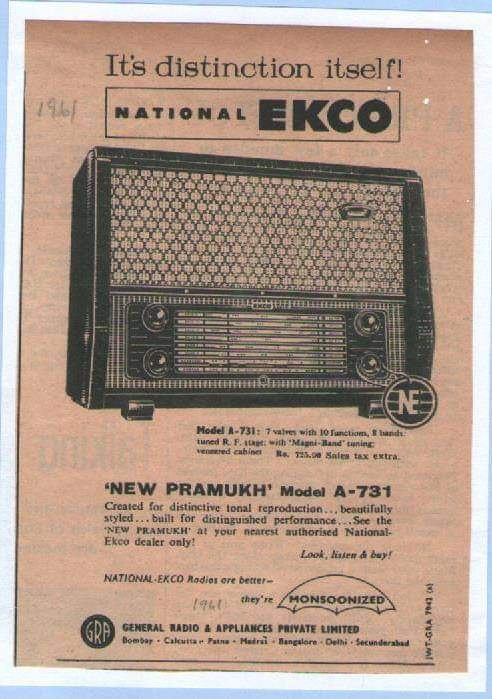This vintage advertisement, appearing like an old newspaper snippet, features a timeworn, taupe-y, orange-brown paper with a pinkish tint, bordered in blue and white. At the top-center in bold black letters, it declares, "It's Distinction Itself!" followed by "National EKCO" and "EKC0." Below, an image of an old radio, identified as the New PRAMUK Model A731, occupies the center. The text highlights its exceptional audio quality: "Created for distinctive tonal reproduction, beautifully styled, built for distinguished performance. See the new PRAMUK at your nearest authorized National EKCO dealer only. Look, listen, and buy - National EKCO radios are better." The ad also boasts that these radios are "monsoonized," symbolized by an umbrella graphic. Scattered across the paper, handwritten in pencil, are the year "1961" inscribed in the top-left corner and repeated at the bottom. The advertisement is concluded by the seal of "General Radio and Appliances Private Limited" at the bottom, symbolized by a circular logo with the letters "GRA."